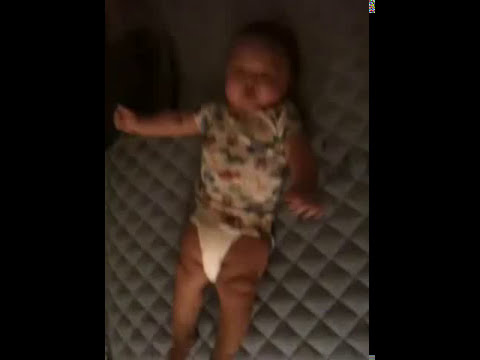This photo shows a baby lying on its back at the center of a blurry, grainy indoor scene, likely captured with an older camera. The baby, dressed in a white top possibly adorned with indistinct dinosaur patterns and wearing a diaper, is positioned on a fabric surface that resembles a quilt or a blanket with linear textures that could be mistaken for a futon. The top and left of the image feature unexplained darker coloring, adding to the vintage and unclear quality. The background fabric displays a variety of colors—gray, tan, white, green, red, yellow, and black—providing a stark contrast to the baby's lighter clothing. The baby gazes upwards, its right arm extended horizontally to the side and its left arm positioned lower and slightly off the fabric. Both legs are stretched out towards the bottom of the photo, although the feet are not visible. No text appears in this image, underscoring its simplistic and timeless nature.